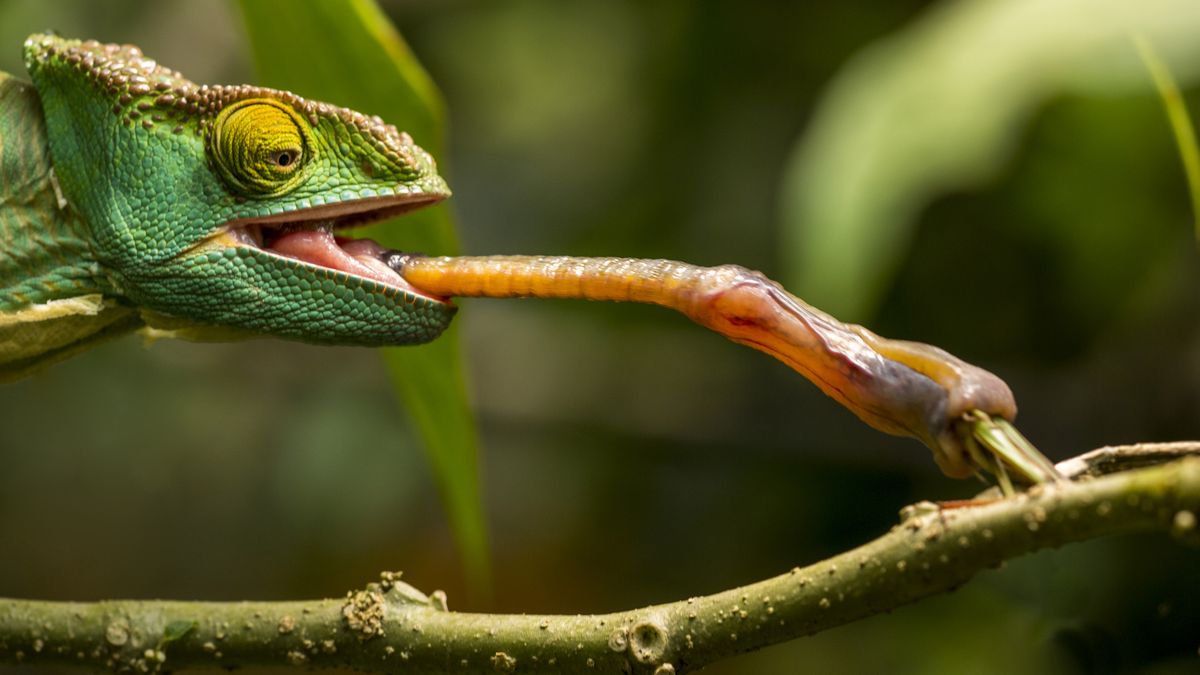The vibrant photograph captures an emerald green chameleon in incredible close-up detail, illustrating its elongated, orange-reddish tongue in the precise act of snaring an insect. The chameleon's head, adorned with bright green scales and striking neon green eyelids, fills the left side of the image, its keen brown eye focused intensely on its prey. The vividly colored reptile's tongue stretches out to nearly twice the length of its head, wrapping around the barely visible legs of the insect. They both perch on a green stem, enveloped in the natural tones of the lush background, which is softly blurred to emphasize the intricate details of the chameleon and its uniquely textured scales. Surrounding foliage, out of focus, hints at a verdant environment, adding further depth to the image.